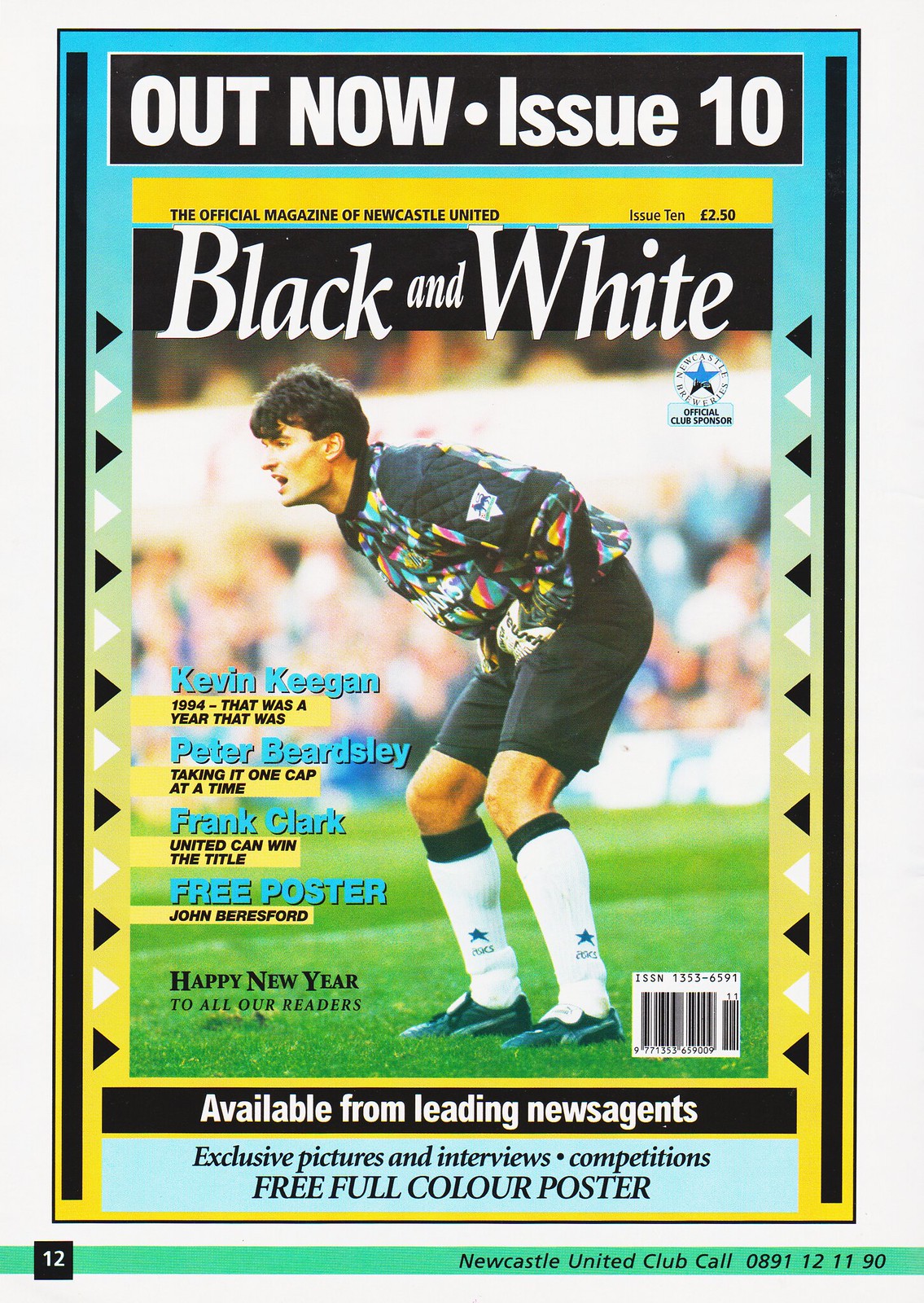The cover of the soccer magazine prominently declares "Out Now Issue 10" on a black bar with white text. Below, a yellow bar with black writing states, "The Official Magazine of Newcastle United, Issue 10, £2.50," and next to it, "Black and White" along with the official club logo. The main image features a man in a colorful, rainbow-patterned shirt with black sleeves, black shorts, white socks with black bands, and black shoes. He is crouching with hands on his upper thighs, pointing slightly to the left, standing on lush green turf. In the blurred background, spectators are visible in the stands.

Headlines in blue include prominent names: "Kevin Keegan - 1994 That Was a Year That Was," "Peter Beardsley - Taking It One Cap at a Time," "Frank Clark - United Can Win the Title," alongside a mention of a "Free Poster - John Beresford," and a greeting, "A Happy New Year to All Our Readers." The bottom part of the cover features a barcode near the man's feet and a black bar stating, "Available from Leading News Agents."

Further highlights in light blue text on a black background include, "Exclusive Pictures and Interviews, Competitions, Free Full-Color Poster." The left and right sides of the cover are bordered by black vertical bars, with a black and white triangle pattern extending from about a third of the way up to a third of the way down the page. The bottom green strip, acting as an additional feature or page footer, includes a white "12" on the left and the inscription, "Newcastle United Club Call 0891-121190," on the right.